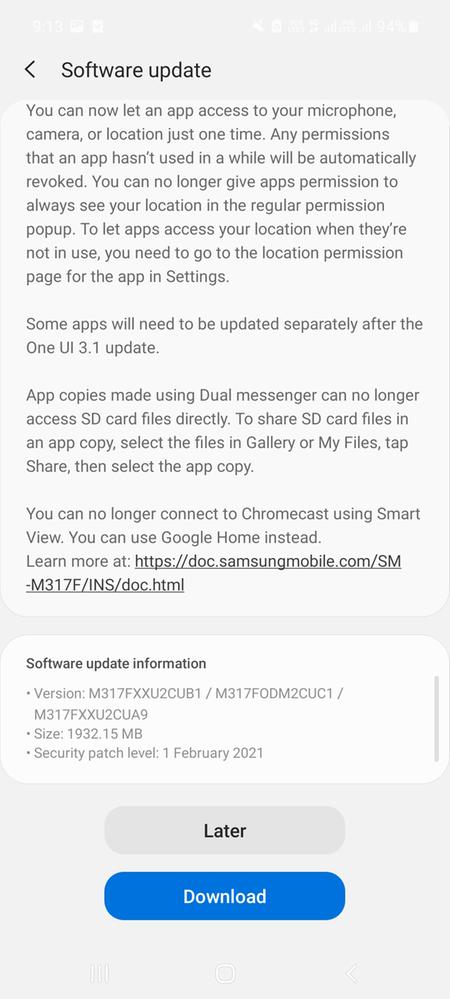The image is a screenshot taken from a cell phone, evident from the visible indicators at the top that display the time, battery at 94%, sound off icon, and other indistinct icons due to a light background. The central focus is a software update notification. 

The notification features an arrow pointing left and the text "Software Update" in bold black font. The information conveyed within the notification includes several key points:

- Users can now grant app permissions for the microphone, camera, or location on a one-time basis.
- Permissions for apps that haven't been used in a while will be automatically revoked.
- The option to allow apps to always access location has been removed from the regular permission pop-up.
- For apps to access location when not in use, users must navigate to the app's location permission page in settings.
- Some apps may require separate updates post the One UI 3.1 update.
- Apps duplicated using Dual Messenger can no longer directly access SD card files. To share SD card files with an app copy, users must select files in Gallery or My Files, tap Share, and then choose the app copy.
- Chromecast connection using Smart View is no longer supported; users can utilize Google Home instead.
- A clickable link for additional information is provided (https://doc.samsungmobile.com-sm-m317f-ins-doc.html).

At the bottom of the screen, there are two buttons, "Later" and "Download," with the "Download" button highlighted in blue.